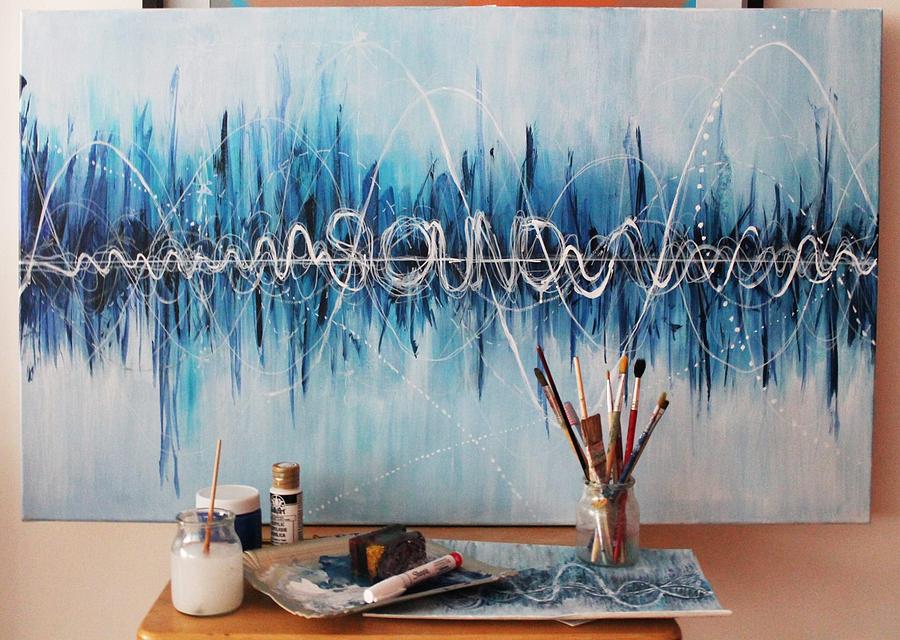This color photograph is a horizontally-aligned, almost square-shaped image capturing an artist's workspace. In the foreground, on a small wooden table, there is a clear glass jar filled with around ten paintbrushes. Nearby, a second glass jar contains a milky white liquid with a paintbrush standing upright in it. Beside it, there is a white and red-tipped Sharpie marker resting on a little tray, which also contains some paint. To the right, there’s a sheet of paper that mirrors the artwork on the wall above.

Dominating the background is a horizontal rectangular canvas painting, hanging on a tan-colored wall. The artwork primarily features various shades of blue, interspersed with a central thin white line. Above and below this line, a series of white sine waveforms are painted, with intricate waves directly on the line spelling out the word "sound." The meticulous details, from the wavy patterns to the scattered art supplies, create a lively and creative scene.